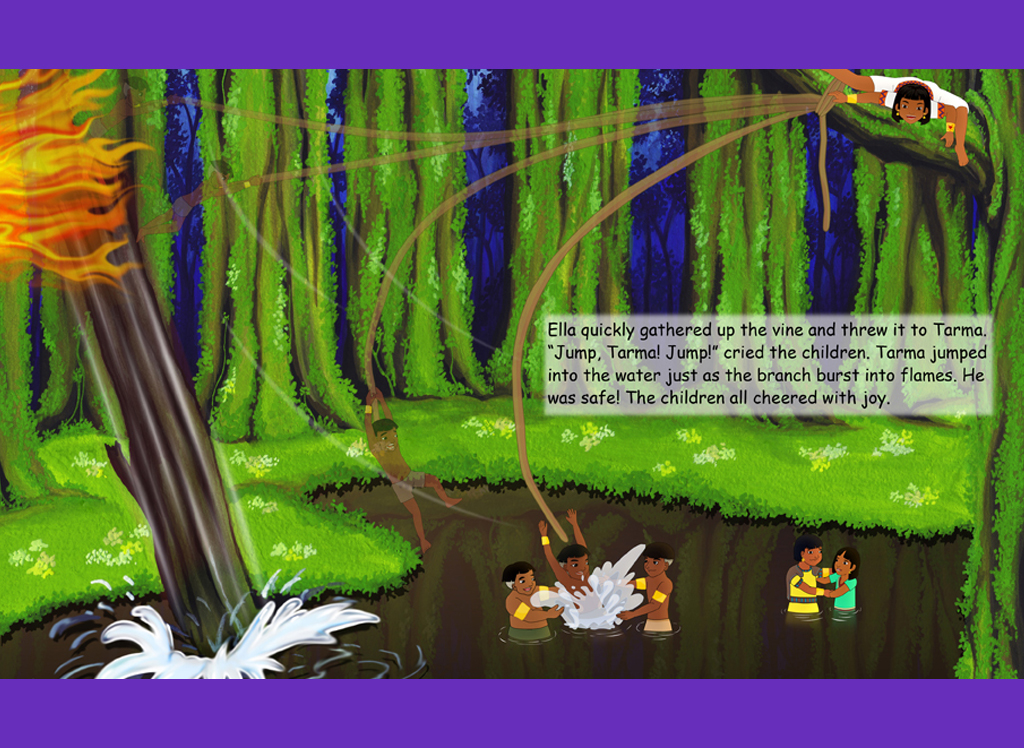This vibrant, single-panel cartoon image, possibly from a comic book or children's story, is brimming with action and detail. Set in a lush rainforest, the background is dominated by towering green-trunked trees wrapped in moss, standing tall around a muddy brown pond. The edges of the panel are bordered in dark purple, adding a framing contrast to the bright central scene. Red flames flicker ominously from the upper left corner of the panel, near a waterfall tumbling into the pond below.

At the heart of the image, lively groups of children are engaged in playful activities in and around the pond. One child swings daringly from a vine, poised mid-air, ready to leap into the water. In the pond, five children, up to their waists in water, seem to be cheering or playing. One child has just made a splashy entrance into the pond, indicated by the white splash around them. Perched on a branch in the upper right corner, another child looks down, adding to the animated atmosphere of the scene.

A horizontal text box on the right center reads: "Ella quickly gathered up the vine and threw it to Tarma. 'Jump, Tarma, jump!' cried the children. Tarma jumped into the water just as the branch burst into flames. He was safe! The children all cheered with joy." This makes it clear that the children are participating in a thrilling rescue scene, filled with excitement and relief.